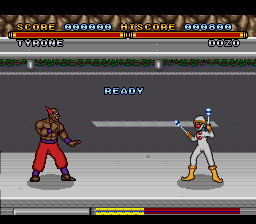This scene is a detailed screenshot from an old-fashioned, cartoon-style fighting video game. Two characters are poised for combat on what appears to be the flatbed of a truck with a steel floor, lined with studs and flanked by various environmental details such as a red and yellow light, a gray bar, green shrubs above, and white lines marking a black asphalt road. 

On the left stands Tyrone, a muscular, bald, black man who is shirtless and dressed in red pants with brown boots. He is in a fighting stance, ready for action. On the right is Dozo, dressed in a white jumpsuit with yellow boots, featuring two prominent red buttons. Dozo resembles a clown with a red nose and clown shoes, holding blue and white glowing maracas. He is also ready to engage in battle.

The screen’s top section displays scores in yellow text: Tyrone’s score at 222,222 on the left and Dozo’s at 222,822 on the right. They have corresponding red health bars. In the center of the screen, "Ready" is displayed in blue, indicating the imminent start of their fight. The background is gray, complementing the steel surface on which the characters stand. A timer bar is visible at the bottom, setting the stage for the showdown.